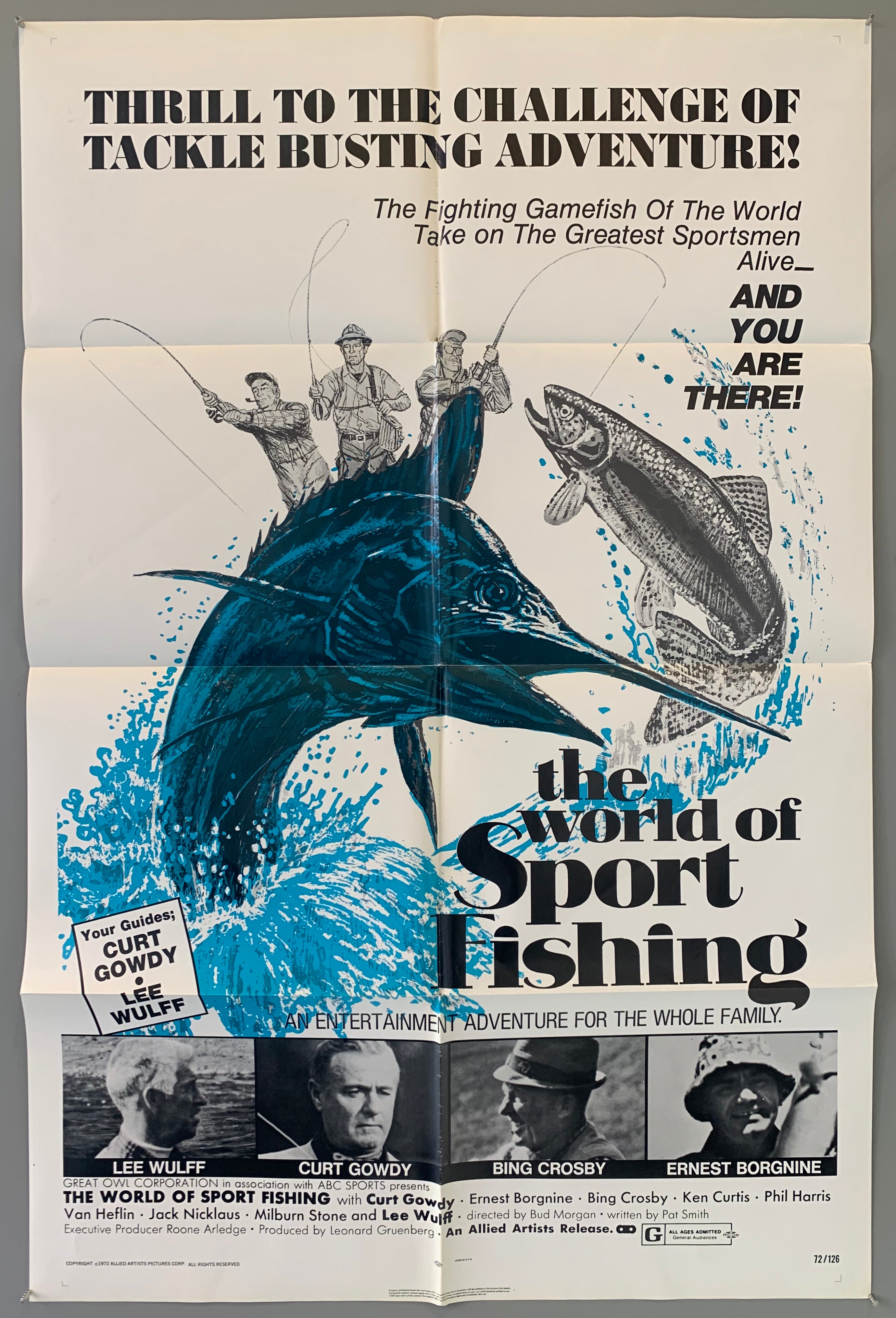The described image is a vintage movie poster specifically promoting a family-friendly documentary about sport fishing. The rectangular poster, which is taller than it is wide, prominently features the headline, "Thrill to the Challenge of Tackle Busting Adventure," introducing the excitement of world-class game fishing. The visual centerpiece is a striking depiction of a blue marlin splashing out of the water, set against an otherwise black and white background. Below this, there's a montage of black and white photos showcasing renowned fishing personalities, including Lee Wulff, Kurt Gowdy, Bing Crosby, and Ernest Borgnine. Additionally, the phrase "The World of Sport Fishing" is boldly printed, emphasizing the documentary's theme. The poster also mentions that it is an entertainment adventure suitable for the entire family, rated G, thus ensuring its broad appeal. Despite some wear evident from fold lines, the overall design effectively captures the thrilling essence of sport fishing and the notable figures associated with it.